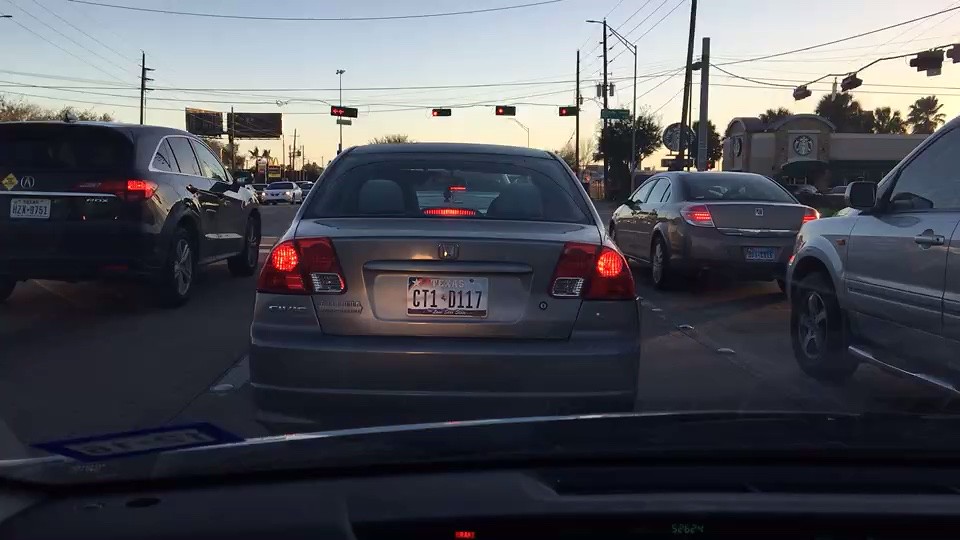The photograph, taken from the driver's seat inside a car, captures the scene of being third in line at a red traffic light on a multi-lane road during dusk, with the gray sky indicating the sun is setting. The gray Honda Civic directly ahead, prominently displaying Texas license plate CT1D117, has its brake lights illuminated. Surrounding the Honda Civic are various vehicles, including SUVs and a pickup truck, all waiting at the intersection. The street is lined with white road markings and cat's eyes, hinting at a suburban environment. To the right of the photo, a Starbucks coffee shop with its recognizable green sign adds a touch of familiarity to the otherwise muted scene. The picture also reveals a small section of the car's windshield and dashboard, enhancing the perspective of being inside the vehicle.